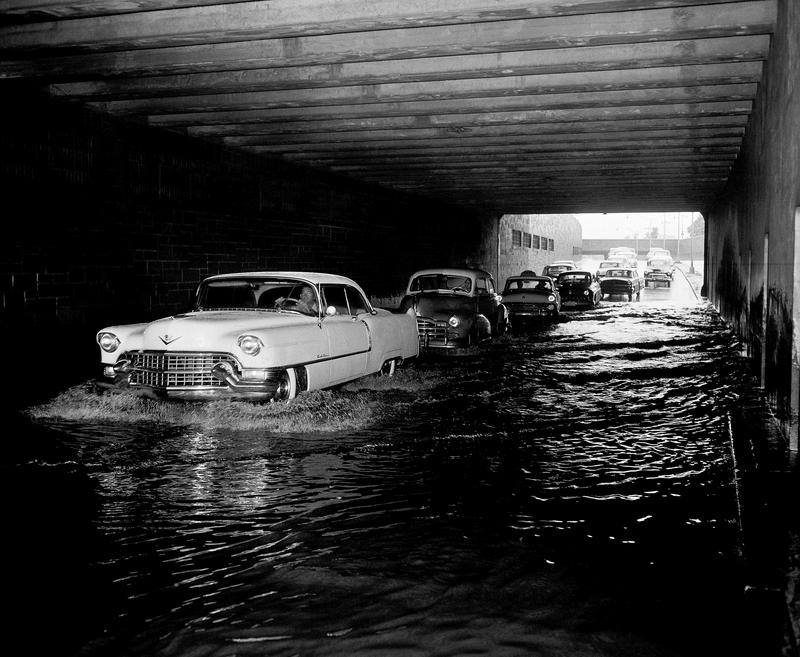This vintage black-and-white photograph captures a striking scene of classic cars, predominantly from the 1940s and 1950s, attempting to traverse a severely flooded highway overpass. In the foreground, a pristine white Cadillac from the 1950s splashes aggressively through the dark, murky waters, leading a procession of about six to seven vehicles following cautiously behind. The water beneath it appears to be six to eight inches deep and rises up dramatically around the wheels of the cars, particularly the Cadillac. The scene sets an evocative image under the arch of the tunnel, with the tunnel's mouth opening toward the center right of the image, revealing daylight and more cars positioned on a slightly higher and dryer part of the road.